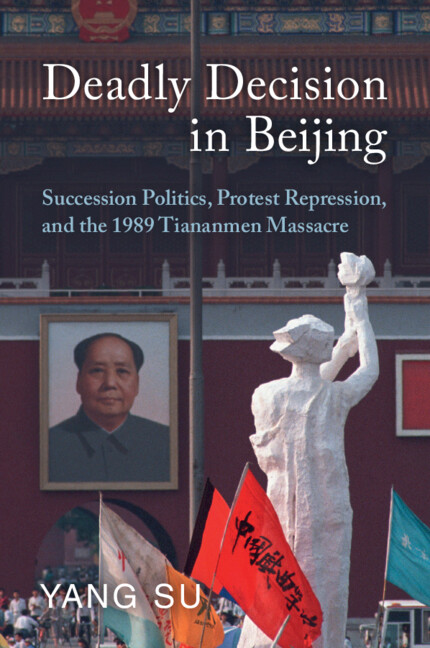This is the cover of a book titled "Deadly Decision in Beijing: Succession Politics, Protest Repression, and the 1989 Tiananmen Square Massacre" by Yang Tzu. The cover features a detailed background of a prominent Chinese building adorned with a large, serious portrait of Mao Zedong under a balcony. In the bottom right corner, there is a stylized, roughly carved white statue of a woman holding up a torch with both hands. Below the statue, several colorful flags in shades of red, orange, and blue with Chinese characters are visibly held aloft. The title and author's name are prominently displayed in white text, with the subtext in light blue. The overall imagery and texts poignantly encapsulate the historical and political gravity of the book's subject matter.